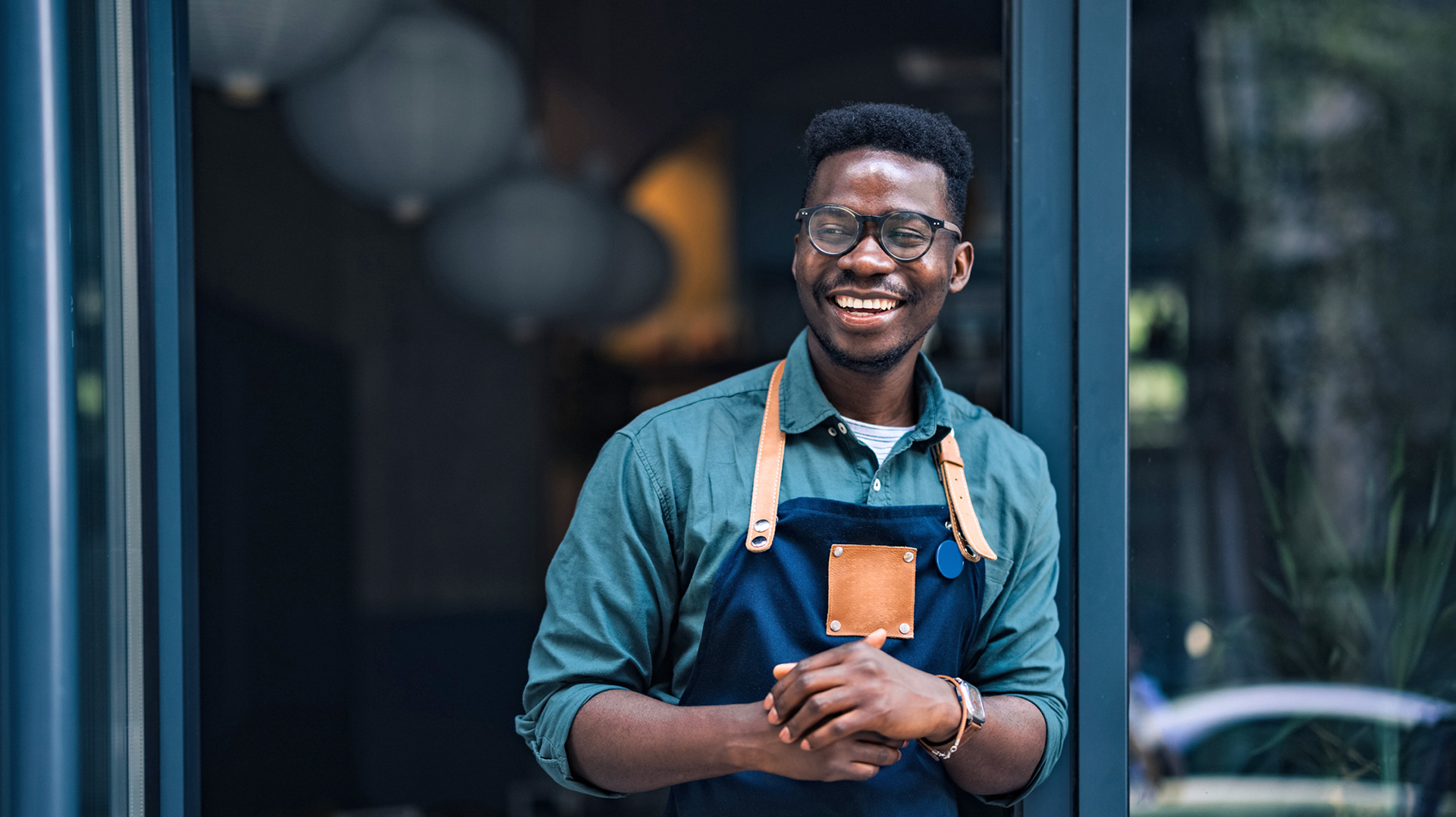This image captures a smiling African gentleman with close-cropped black hair and large, round-framed black glasses. He is dressed in a tealish turquoise button-up shirt with the top button open, revealing a white undershirt, and his sleeves are rolled up to expose his forearms and a watch on his left wrist. Over his shirt, he wears a navy blue apron with a leather strap around his neck and a leather patch on the front, secured by four gold-colored rivets. The background features a slightly translucent, light blackish-gray screen door, through which we can glimpse a restaurant interior with at least three to four white, lantern-like lights hanging from the ceiling.